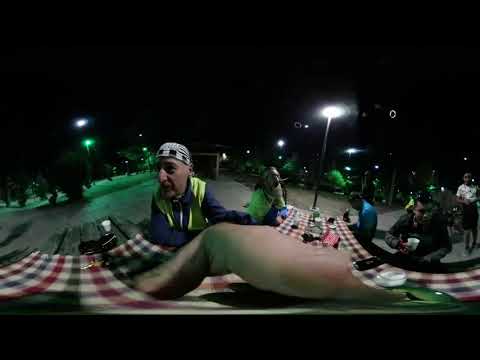In this heavily distorted 360-degree panoramic nighttime image, we find ourselves at an outdoor eating venue, possibly near food trucks. The scene centers around a middle-aged man, distinguishable by his gray mustache and goatee, wearing a black and white bandana on his head. His attire includes a blue long-sleeved shirt and a yellow vest. He is controlling the camera, creating a visual where his outstretched hand in the center appears larger and slightly deformed due to the panoramic distortion. The man is seated at one end of a picnic table adorned with a red, green, and white checkered tablecloth. 

Behind him, two other men sit; one has a long white beard, wearing an outfit similar to the man with the camera, while the other two men are clothed in different shades of blue and green. Alongside them, there are a few more individuals visible, including a person in a white shirt and black skirt, who could be a waitress. The backdrop features streetlights casting a gentle glow over the scene, with trees lining this concrete area. Black horizontal bars frame the top and bottom of the image, possibly as a border. The photograph's dark background indicates the night sky, punctuated by lit streetlights, enhancing the lively atmosphere of this outdoor dining experience.